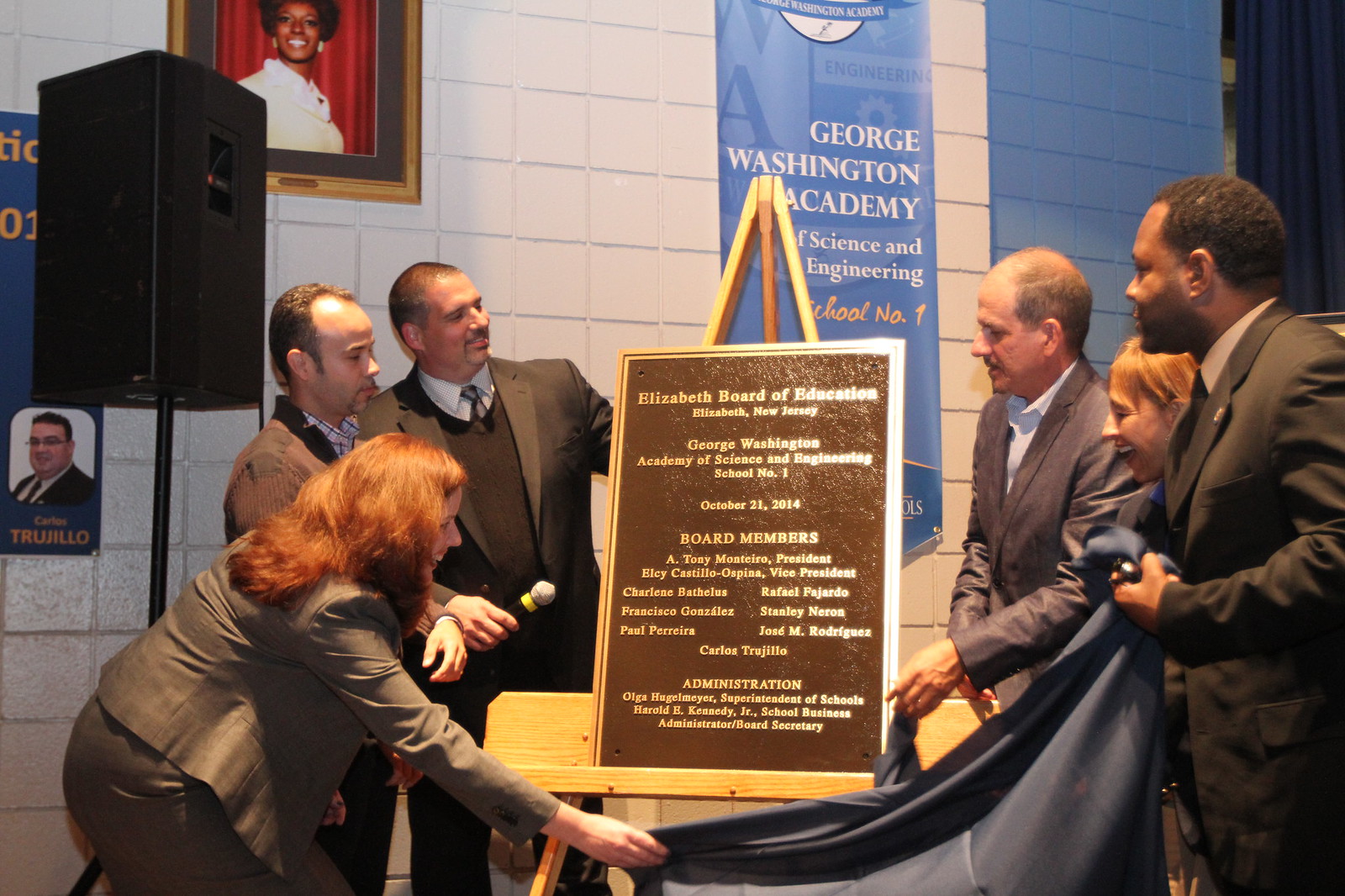The photograph, taken indoors, captures the formal unveiling of a plaque commemorating an event at the George Washington Academy of Science and Engineering, School No. 1, in Elizabeth, New Jersey, dated October 21, 2014. The central focus of the image is the plaque, mounted on a wooden easel, with gold text on a black background. The plaque reads: "Elizabeth Board of Education, Elizabeth, New Jersey, George Washington Academy of Science and Engineering, School No. 1, October 21, 2014." Below this, it lists Board Members: A. Tony Monteiro, President; Elsie Castillo Ospina, Vice President; Charlene Bathillis; Rafael Fajardo; Francisco Gonzalez; Stanley Neron; Paul Perela; Jose M. Rodriguez; Carlos Trujillo. It also lists Administration names: Olga Hugenmeier, Superintendent of Schools, and Harold E. Kennedy, Jr., School Business Administrator/Board Secretary. 

Surrounding the plaque, a group of individuals dressed in formal business attire, including shirts, ties, and suits, stand on both the left and right sides. Positioned in the bottom corners of the image, a man on the right and a woman on the left are holding a blue drape, actively unveiling the plaque. The background features a white brick wall adorned with banners and photographs. One prominent banner reads "George Washington Academy" in blue text, adding context to the setting.